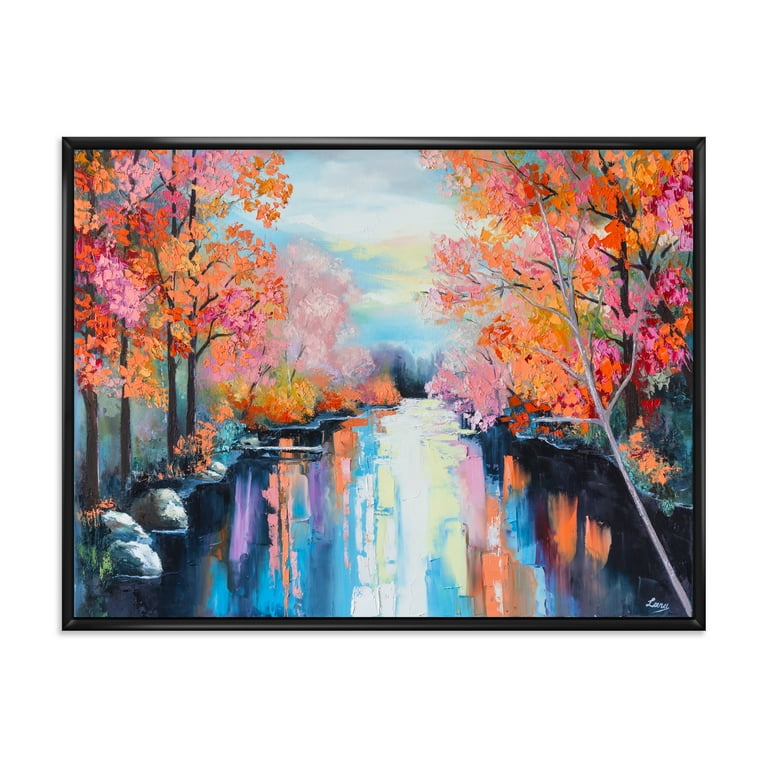This vibrant painting, enclosed in a faint black frame, captures a serene autumn scene where a colorful stream flows through a lush forest. The water, with a blue base, mirrors the vivid hues of the surrounding trees, amplifying the already rich palette. On the left, trees adorned with leaves in shades of orange, red, pink, and yellow fill the foreground, extending to reveal more trees in yellow and green hues. Nestled among these is a singular pink tree, standing out at the back. To the right, a white birch tree leans over the water from the bottom corner, its branches mingling with trees bearing similar fall colors, primarily orange, red, and pink. The bottom left corner of the image also features a few rock-like formations. Overhead, a majority pale blue sky, streaked with white clouds and hints of yellow, hints at the tranquility of the scene. In the background, soft hills and additional trees form a muted but essential part of the landscape. The painting is subtly signed in white at the bottom right corner, adding a personal touch to this exquisite depiction of nature in its autumnal glory.